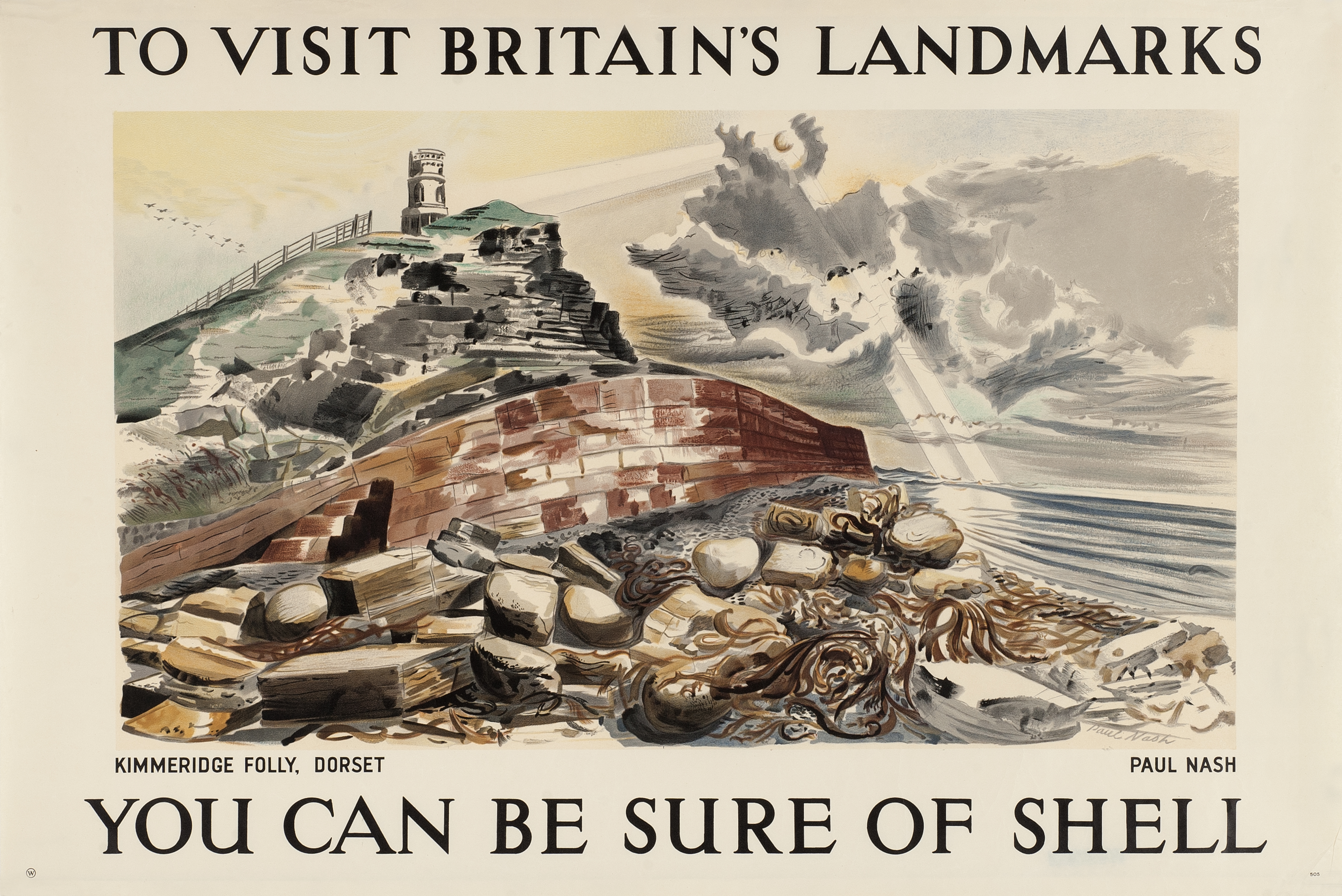This old promotional poster for visiting Britain features a watercolor image centered on a lighthouse atop a hill. The background is a light tan, and the primary text at the top, in medium brown capital letters, reads "TO VISIT BRITAIN'S LANDMARKS." Below the illustration, in similar brown capital lettering, it says, "YOU CAN BE SURE OF SHELL," apparently promoting the Shell company.

The painted image depicts a hillside crowned by a lighthouse with a long, brown stone retaining wall or breakwater near its base. The foreground shows a rocky beach scattered with debris including large rocks, seaweed, and possibly a rope. Behind this, the ocean extends to the right, beneath a stormy sky filled with gray clouds and two white rays of sunlight breaking through. The top left of the image has seven bird-like splotches, portraying seabirds.

In smaller text, the lower left corner of the picture reads "KIMMERIDGE VALLEY DORSET," while the lower right is marked with the name "PAUL NASH," indicating the artist. The scene's primary colors are brown, white, light green, yellow, and gray, evoking a muted, vintage atmosphere.